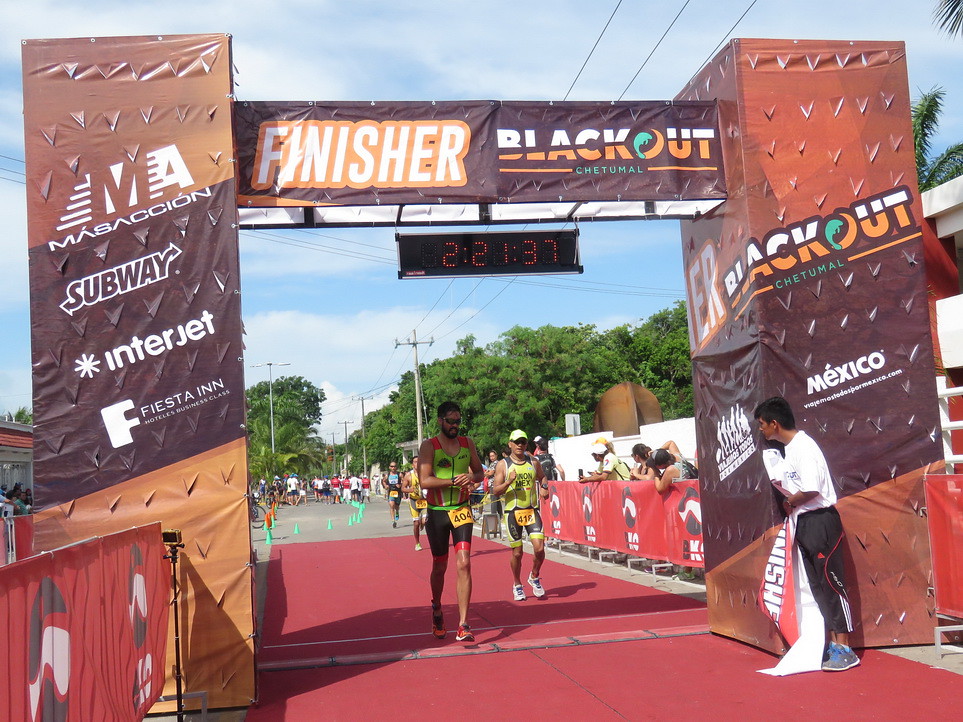The image depicts the dramatic finish line of a race set in a square under a structured archway. Two prominent male runners are in the spotlight as they dash towards the finish line. The leading runner, a tall man adorned in neon green shorts and sunglasses, sports a number 404 on an orange tag affixed to his thigh. His dark brown beard and hair are visible, with his arms positioned in front of him. Trailing closely behind him on the right is another competitive runner wearing a bright neon yellow cap and a similarly colored shirt, bearing the number 418 in black letters on another orange tag. He is dressed in matching yellow and black shorts and white trainers, complemented by sunglasses.

Above them, a digital timer glows in orange dots, displaying the time '2:21:37' against a black background. Accompanying the scene are two towering columns flanking the finish line, adorned with various logos including Master Sion, Subway, Interjet, and Fiesta Inn on the left column and Blackout, and Chet-A-Mole on the right. A 'Finisher' banner stretches across the center of the archway, marked in white letters outlined in orange.

In the periphery, a man in a white polo shirt and black trousers holds a rolled-up banner, observing the racers with keen interest. Behind him, spectators line the fenced pathway, protected by plastic sheeting, as they cheer on the contestants. The clear blue sky dotted with patches of white clouds provides a serene backdrop, juxtaposed against the electrifying energy of the race. In the far distance, more runners with yellow tags approach the finish, while lush green trees frame the entire scene, adding a natural touch to this momentous event.